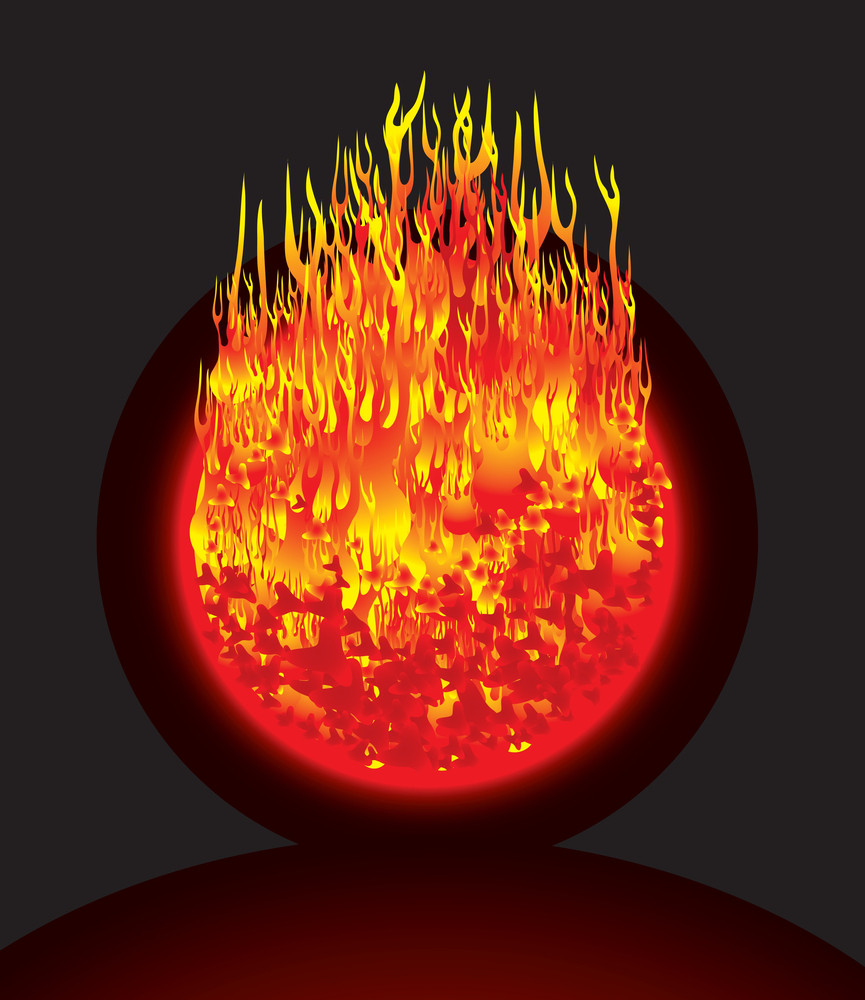The image depicts a striking 3D illustration of a luminous fireball, meticulously centered against a dark, textured background. Dominating the composition is a black, circular orb which houses a brilliant, multi-hued conflagration of flames in vibrant shades of yellow, orange, and red. These flames exude a dynamic, upward thrust, extending beyond the orb's boundaries and creating a vivid contrast against the surrounding darkness. The core of the orb glows intensely, featuring a red, molten center that adds depth to the fiery visual.

Encapsulating the flames is a deep black ring, even darker than the encompassing dark hues of the background, which imparts an almost enigmatic quality to the piece. Below the primary orb, there is a slight, intriguing glimpse of what appears to be another sphere, suggesting a layered, celestial narrative—perhaps a meteor in descent or an abstract, cosmic collision. These elements contribute to a sophisticated geometric design, accentuated by the neon-like luminance of the flames, making the artwork both captivating and thought-provoking.